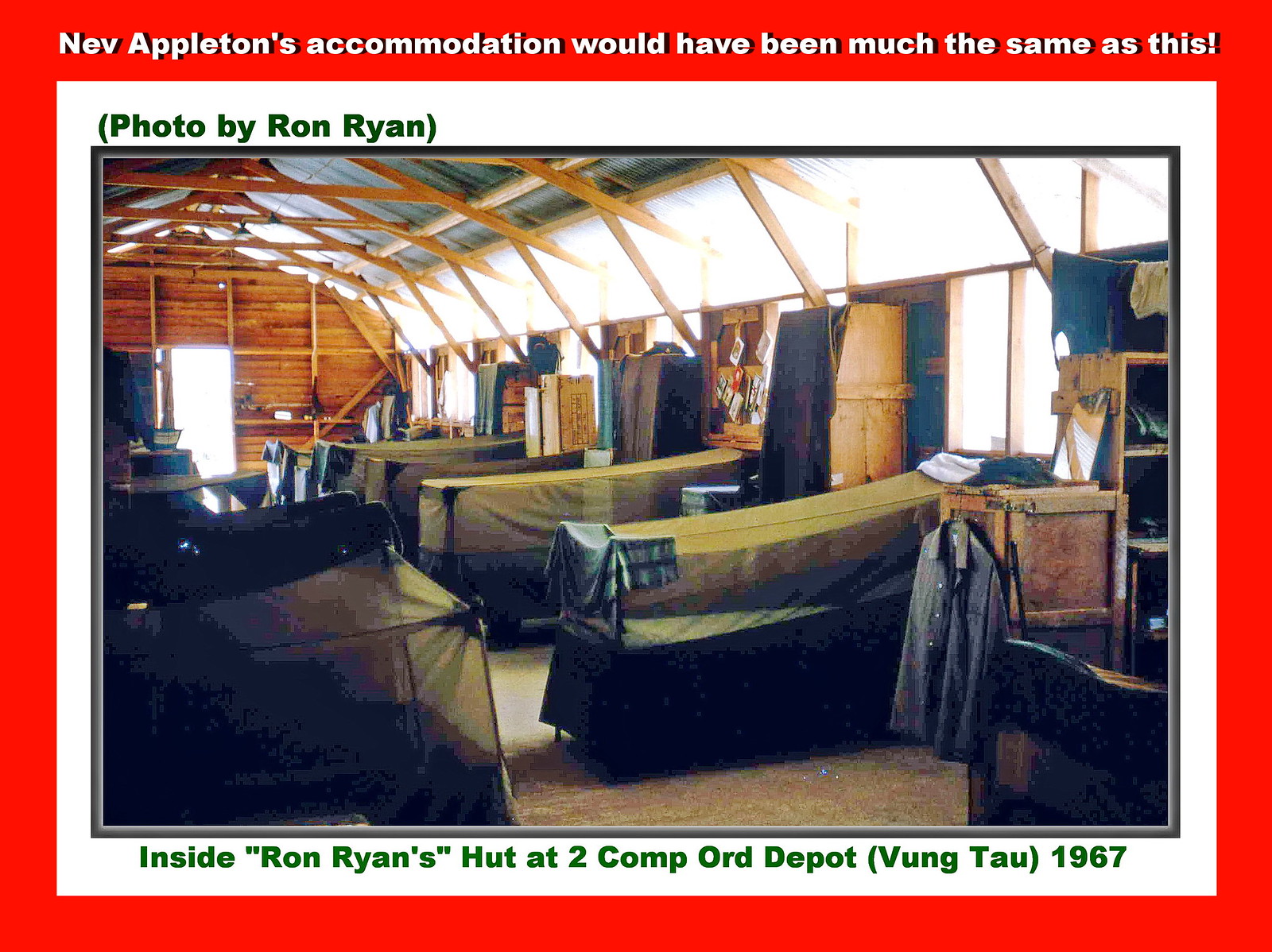This detailed rectangular image features a digitally composed frame with two layers. The outer frame is bright red, with white text at the top reading, "Nev Appleton's accommodation would have been much the same as this!" Inside the outer frame, a white inner frame appears with green text at the top in parentheses stating, "(photo by Ron Ryan)." The bottom of the inner frame bears a green caption: "Inside Ron Ryan's hut at Two Comp or Depot, Vung Tau, 1967."

At the center of this framed image, a photograph captures a cabin with a green, triangular ceiling. Within the cabin, multiple beds equipped with bug nets are meticulously arranged in rows, lining both sides of the space. This photograph exudes a sense of sparse military accommodation, suggesting the utilitarian and cramped conditions the inhabitants experienced. Despite its simplicity, the image reveals intricate details of a living space that once provided shelter and some degree of comfort amidst a challenging environment.